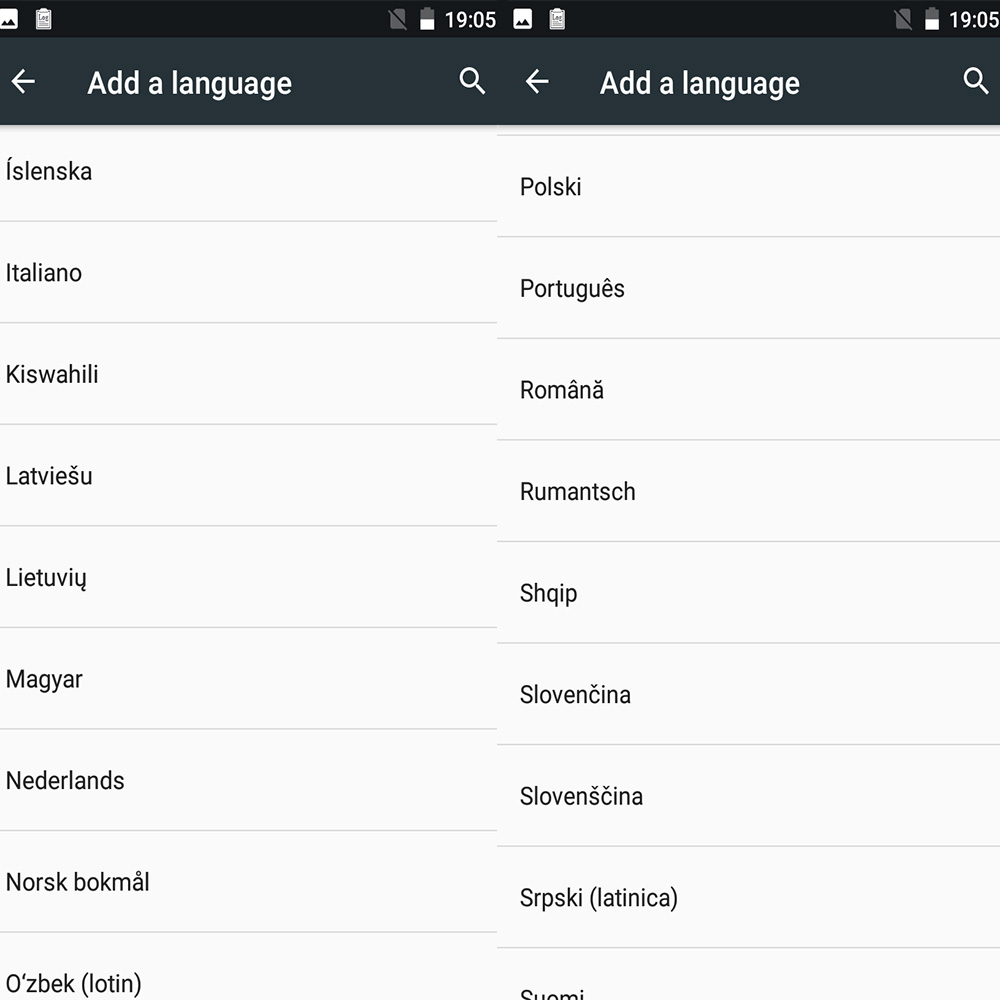Two side-by-side screenshots display the settings of an Android smartphone used in landscape mode. Both screenshots reveal a black bar at the top, which contains a "Back" button and the text "Add a language". The phone is operating without a SIM card, as indicated by the lack of signal, and the battery level is at 50%. The screenshots were taken on the 5th of January. 

The left screenshot shows a list of languages available for addition, including Icelandic (Íslenska), Italian (Italiano), Kurdish (Kurdî), Swahili (Kiswahili), Latvian (Latviešu), Lithuanian (Lietuvių), Hungarian (Magyar), Dutch (Nederlands), Norwegian Bokmål (Norsk bokmål), and Ossetic (Осетинский). Meanwhile, the right screenshot features another set of languages: Polish (Polski), Portuguese (Português), Romanian (Română), Russian (Русский), Albanian (Shqip), Slovenian (Slovenščina), Slovak (Slovenčina), and Serbian (Српски, Latinica). At the bottom of this list on the right side, there is a barely visible option for the Somali language (Soomaali). 

These screenshots capture the user's activity as they navigate through the language settings on their Android device, attempting to add a new language to the system.